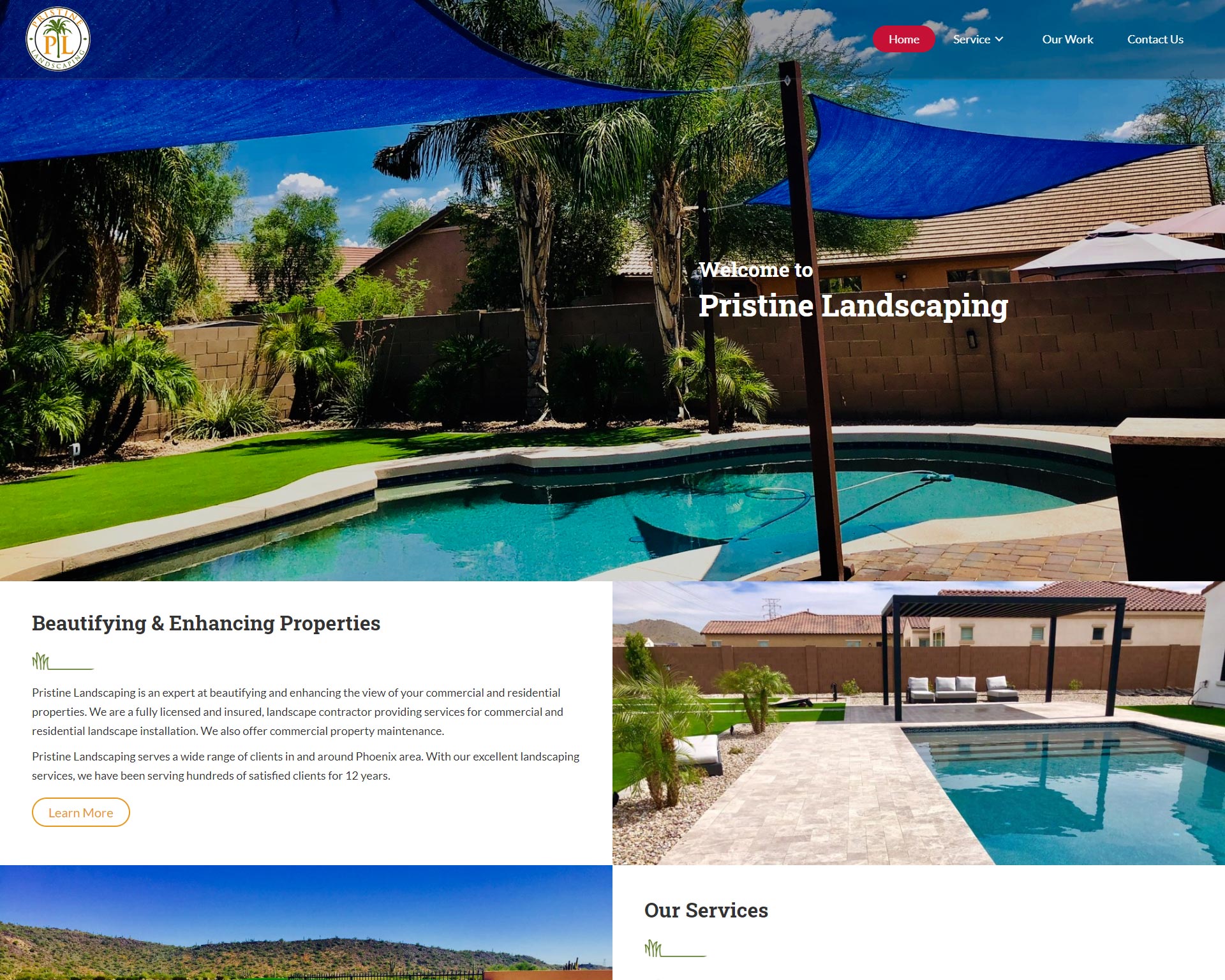A stunning pool area featuring a unique design with triangular blue canopies providing ample shade. The pool is framed by verdant green grass and bordered by stately palm trees. Adjacent to the pool is a charming building with a brown roof and matching brown walls. On the far end of the pool, a black cover offers additional shade, beneath which white chairs are placed for relaxation. The backdrop includes a picturesque blue sky, lush green bushes, and rolling hills, creating a serene and inviting atmosphere. Experience the perfect blend of home and nature. Contact us to learn more about our services in enhancing and beautifying properties.